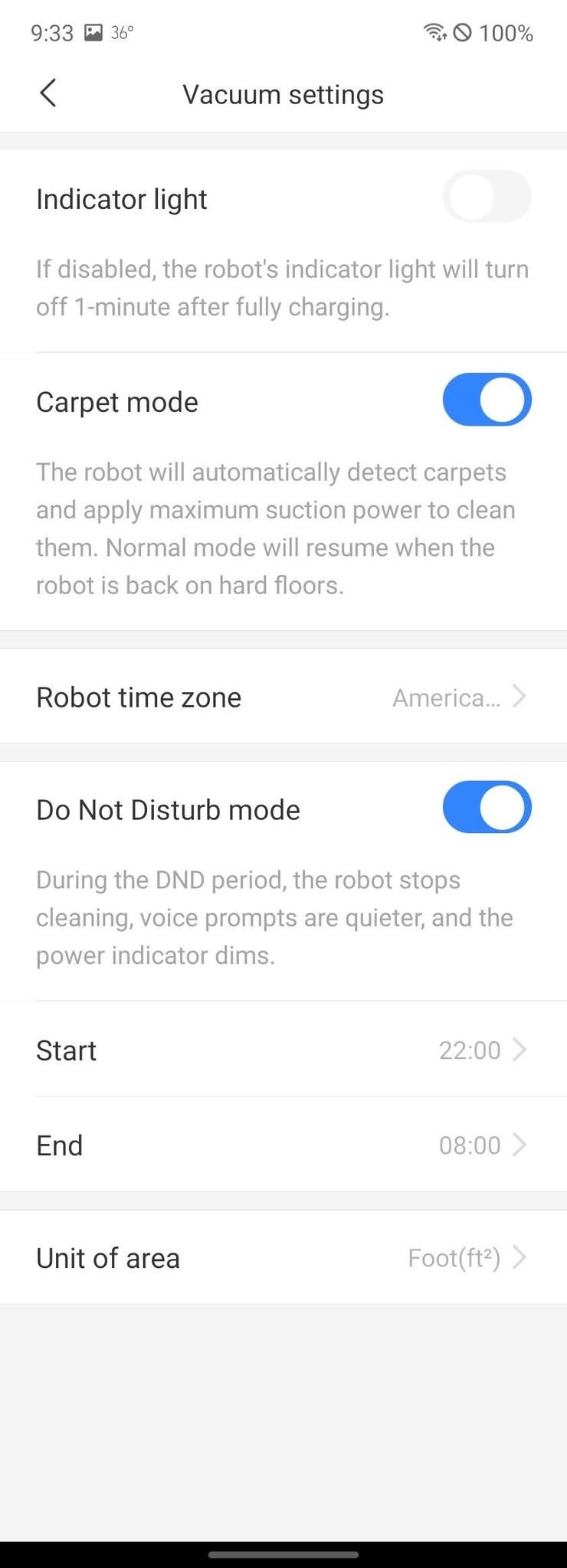Screenshot of a smart vacuum cleaner interface in portrait mode on a white background. 

**Top Left Corner:**
- Time: 9:33
- Temperature: 36 degrees

**Top Right Corner:**
- Battery: 100% charged

**First Row:**
- Back arrow
- Vacuum settings

**Second Row:**
- Toggle Switch (Off)
- Label: "Indicator Light"
- Description: "If disabled, the robot's indicator light will turn off one minute after fully charging."

**Third Row:**
- Toggle Switch (On)
- Label: "Carpet Mode"
- Description: "The robot will automatically detect carpets and apply maximum suction power to clean them. Normal mode will resume when the robot is back on hard floors."

**Fourth Row:**
- Label: "Robot Time Zone"
- Value: "America"

**Fifth Row:**
- Toggle Switch (On)
- Label: "Do Not Disturb Mode"
- Description: "During the DND period, the robot stops cleaning, voice prompts are quieter, and the power indicator dims."

**Sixth Row:**
- Start Time: 22:00
- End Time: 08:00

**Seventh Row:**
- Label: "Unit of Area"
- Value: "Square foot"

**Summary:**
This interface is for a programmable AI-enabled robovac, allowing users to configure various settings such as indicator lights, carpet mode, time zone, and Do Not Disturb mode through an app.